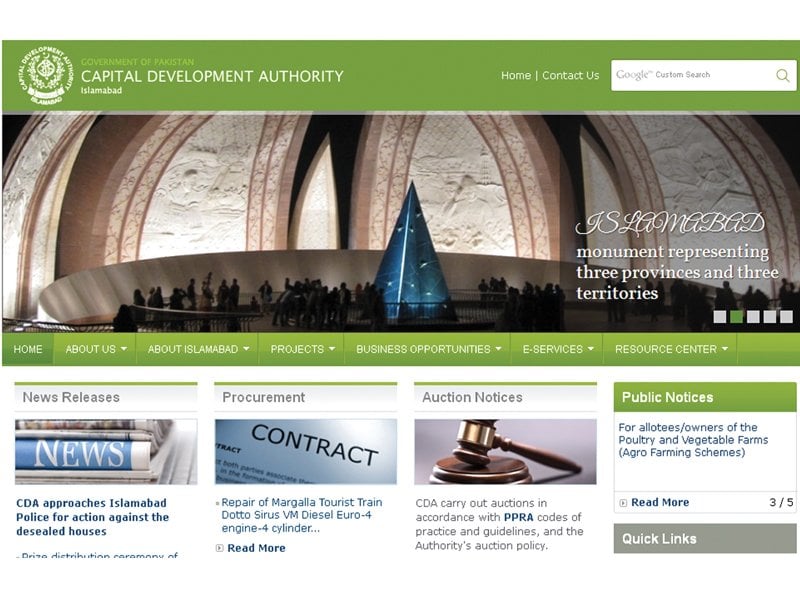**Image Description:**

At the top of the image, the heading "Capital Development Authority" is displayed in green, followed by "Government of Pakistan Islamabad." An intricate logo featuring a wreath and the text "Capital Development Authority" is situated next to this heading. To the right of the logo, there are navigation options labeled "Home," "Contact Us," and a white search box with a magnifying glass icon, indicative of a Google custom search function.

Beneath the header, the image showcases a prominent blue triangular structure framed by leaning walls, with numerous silhouetted figures at the bottom, indicating the site's bustling activity. A caption reads "Islamabad Monument representing three provinces and three territories."

Below this main image, several green tabs provide navigational links: "Home," "About Us," "About Islamabad," "Projects," "Business Opportunities," "E-Services," and "Resource Center." 

Further down, there's a section titled "News Releases" accompanied by a newspaper icon. Below are updates, including "CDA approaches Islamabad police for action against the de-sealed houses." 

Next to it, under "Procurement," one finds "Contract." Adjacent to this, "Auction Notices" mentions "CDA carry out auctions in accordance with PPRA codes of practice and guidelines and the authority's auction policy." 

Additionally, a section labeled "Public Notices" contains pertinent announcements. Finally, at the bottom right of the image, a segment titled "Quick Links" is available for rapid navigation.